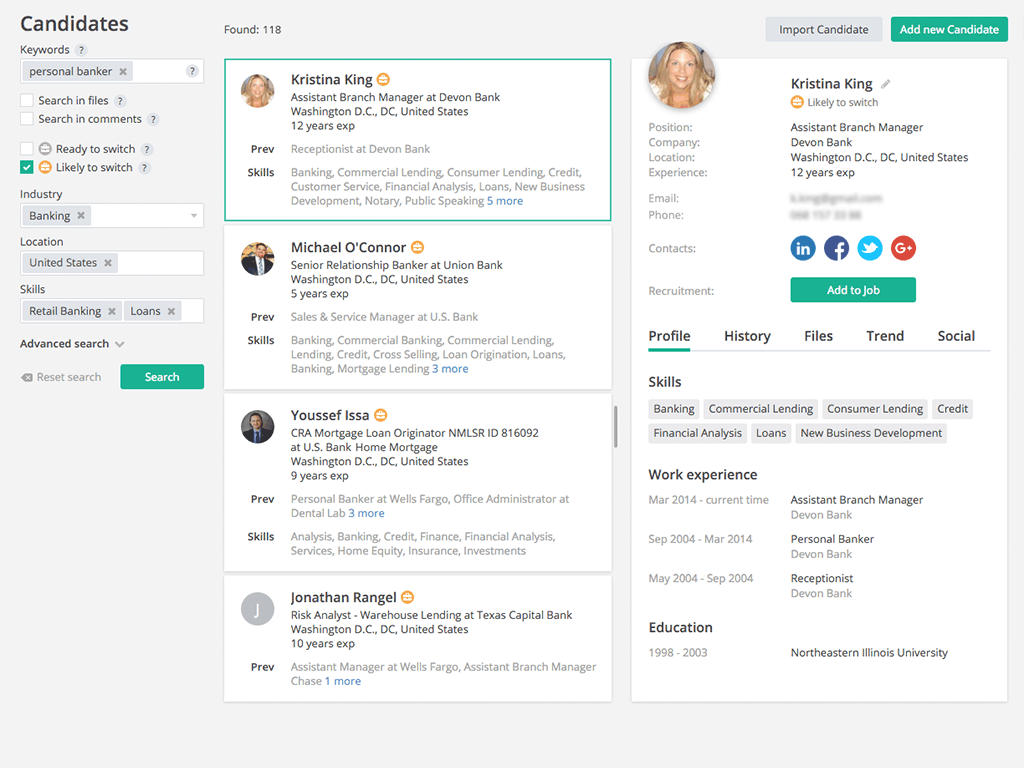The screenshot showcases a digital candidate profile interface against a light gray background. In the upper left corner, the word "Candidates" is prominently displayed in bold black text, with a smaller gray text to its right indicating "Found 118." On the upper right, there are two clickable boxes: a gray "Import Candidate" box and a green "Add New Candidate" box.

Directly beneath the "Add New Candidate" box, another section of the screenshot features a circular profile image of an attractive blonde woman with fair skin. To the right of her image is the name "Christina King" in bold text, accompanied by a label "Likely to Switch." Her position is listed as "Assistant Branch Manager" at "Devin Bank," located in "Washington DC, DC, United States." She boasts "12 years of experience."

Below her profile name, there's an underlined section titled "Skills," detailing her proficiencies which include: "Banking, Commercial Lending, Consumer Lending, Credit, Financial Analysis, Loans, and New Business Development." Further down, her work experience is summarized: From March 2014 to the current date, she has been serving as "Assistant Branch Manager" at "Devin Bank."